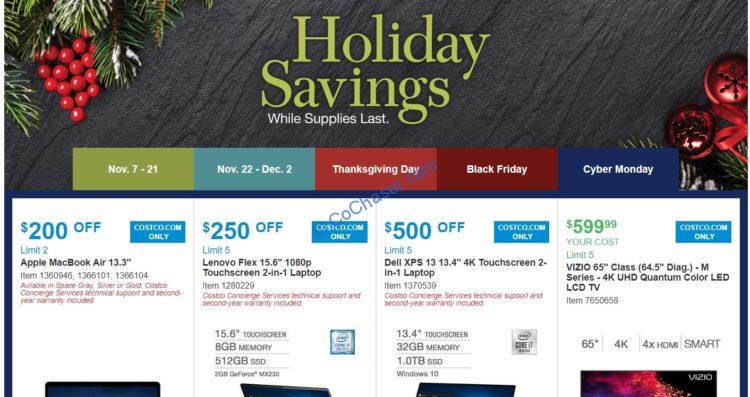This website screenshot showcases a promotional banner for holiday savings. The top of the image features the headline "Holiday Savings" in bold, greenish-yellow text, with a white subtext beneath it that reads "While supplies last." The majority of the background is gray, complemented by a partial wreath in the top left corner and red ornaments on the right.

The image is organized into five rectangular categories, each in alternating colors:
- The leftmost category is green and states "November 7th through 21."
- The next category to the right is light blue, labeled "November 22nd through December 2nd."
- The central category is pinkish-red, marked "Thanksgiving Day."
- To the right of that is a dark red category labeled "Black Friday."
- The far-right category is blue and reads "Cyber Monday."

Below these categories are four discounted deals, each highlighted with text in varying colors:
1. On the far left, "$200 off" in blue text for the Apple MacBook Air 13.3, available exclusively at Costco.com.
2. Next, "$250 off" in black text for the Lenovo Flex touchscreen 2-in-1 laptop, with additional specifics listed below.
3. The third deal offers "$500 off" on a Dell XPS touchscreen 2-in-1 laptop.
4. The final deal is priced at "$599.99" for a Vizio 65-inch flat-screen LED LCD TV.

This detailed layout provides a comprehensive overview of the promotional offers available for the holiday season.